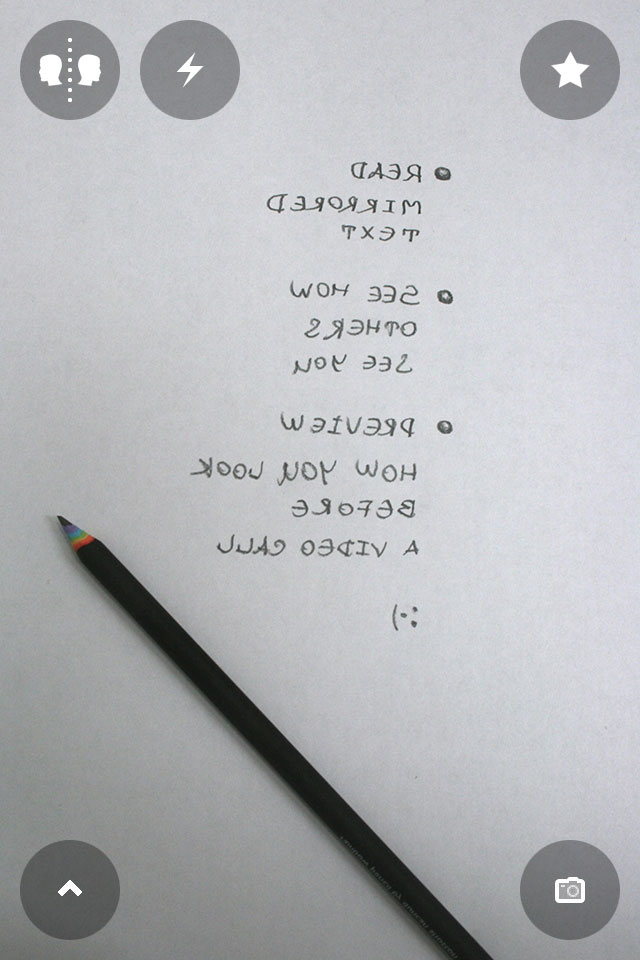The image shows a predominantly gray rectangle with various graphical elements and text. At the very top on the left side, there is a gray circle featuring a white head silhouette on one side, separated by a vertical dotted line, and a white head silhouette on the other side. Adjacent to this is a dark circle containing a lightning bolt symbol.

In the top right corner, there is a dark gray circle with a white star in the center. Below this, written in mirrored dark gray text that needs to be read from right to left, it says "read mirrored text" with a black dot preceding the word "read." Further down, it reads "see how others see you," also with a black dot in front of the word "see," and this text is located on the right side. 

The last section of text, forming a paragraph, says "preview how you look before a video call," accompanied by a sideways smiley face emblem. From the bottom right corner extending diagonally towards the middle left, there is a black pencil featuring a black tip and blue, yellow, and red colors visible from where it has been sharpened.

At the very bottom of the page, there are two dark gray circles: the one on the left contains a triangle resembling a mountain peak without the bottom line, while the one on the right has a white camera icon inside.